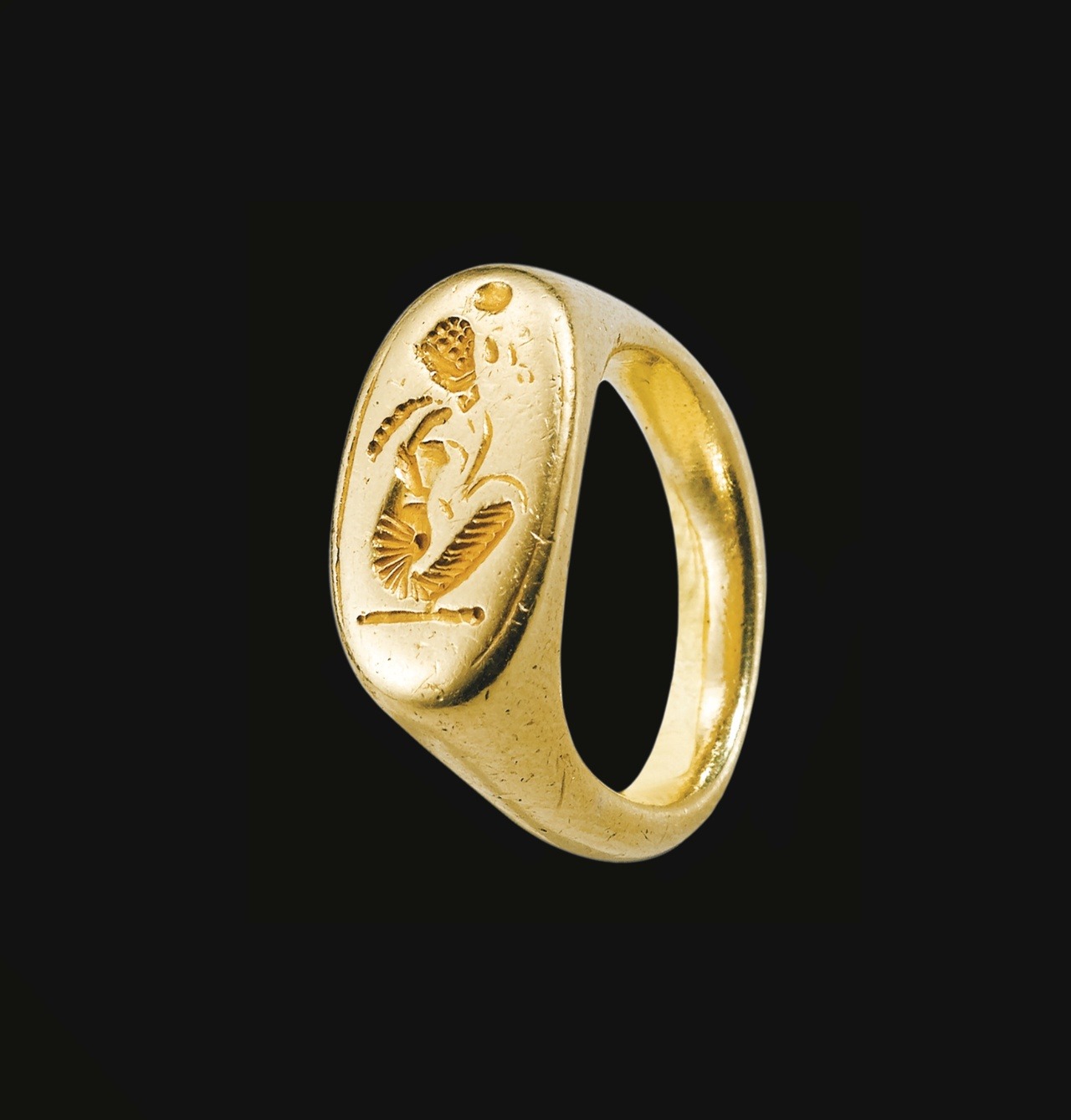This detailed color photograph presents a worn and ancient gold ring set against a completely black background. The image is square, approximately five to six inches on each side. The ring, positioned slightly tilted towards its side, measures about two to three inches in height and one and a half to two inches in width. The gold surface displays clear signs of age, with noticeable pitting, rub marks, and imperfections, suggesting prolonged use.

The flat face of the ring features intricate, engraved designs that include multiple abstract shapes. At the top, there is an indented circle resembling a skull. Below this, a series of fragmented pieces that taper downwards evoke the appearance of elongated string beans. These segmented lines continue and evolve into a U-shaped step pattern, further adding to the elaborate detail. Another similar string bean figure traverses horizontally at the bottom of the design.

Although the exact depiction is worn and somewhat ambiguous, with some interpretations hinting at an abstract portrayal of objects or creatures, the overall craftsmanship indicates the ring might have been used as a seal or stamp. The darkened engravings stand out against the bright yellow gold, enhancing the contrast and detailing of this intriguing artifact.